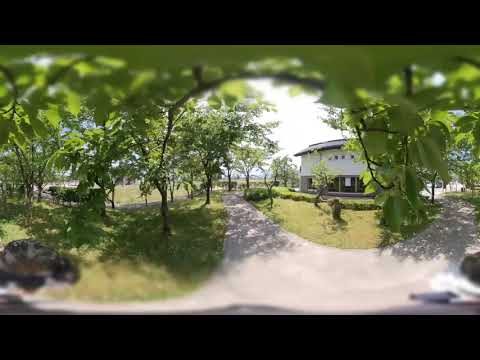This outdoor photograph, with a panoramic distortion and a curved rectangular shape, captures a tranquil scene shrouded in a slight blur. The image is framed by black bands at the top and bottom, emphasizing its unique format. The setting suggests a picturesque yard with meticulously manicured green grass and concrete pathways meandering through the scene. Tall trees with green leaves and brown trunks line both sides, their branches forming a leafy archway over the pathway, adding a touch of natural elegance. 

In the background stands a white building with a sturdy gray base and dark windows, crowned with a black or gray roof. The structure is partially obscured by tree branches and leaves hanging down in front. The sky above, laden with clouds, appears a light gray, casting a bright but subdued light over the scene. The overall atmosphere is serene and devoid of people, giving it a peaceful, almost untouched feel. The grass, shrubs, and strategically placed rocks add to the scenic charm, framing the house with a natural boundary and reflecting the careful landscaping.